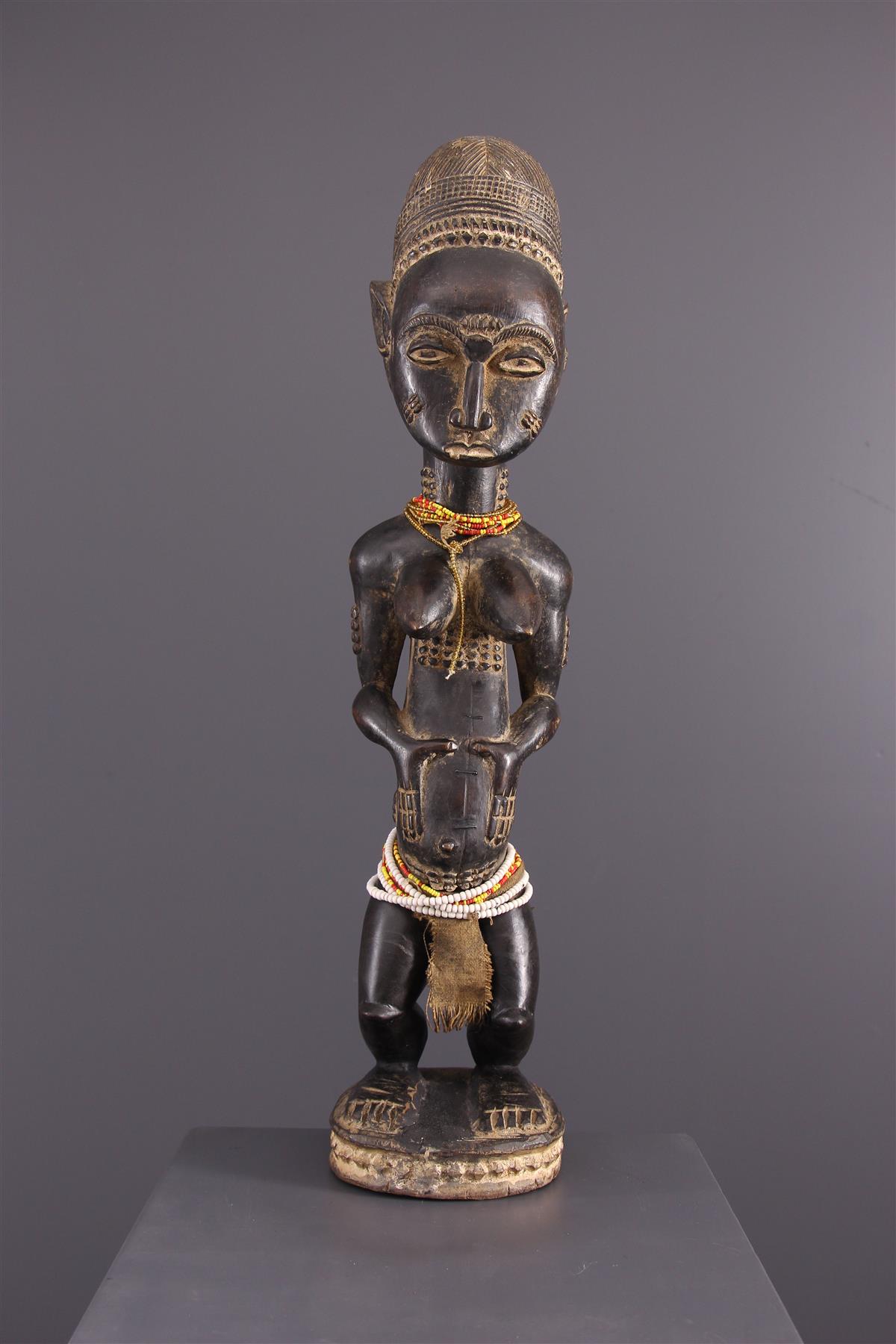The image showcases a detailed, primitive-style metal sculpture that appears to be an African artwork. The sculpture, adorned in hues of deep burnished dark brown, depicts a slightly ambiguous human figure, likely a woman, with exaggerated features. She stands barefoot on a circular base, positioned against a gray background as if being photographed for a listing. The figure is adorned with colored beads - yellow and green beads drape around her neck, and white, yellow, and red beads encircle her waist. She has tribal marks on either cheek, probably signifying cultural importance. The sculpture also features a large headdress or hat, a thick neck, and muscular shoulders and arms. With her hands resting on a protruding stomach, the sculpture suggests she might be pregnant. Her torso is elongated, while her legs are short, stocky, and muscular, ending in wide, flat feet. The artistry captures a blend of strength and cultural symbolism, making it a striking piece.